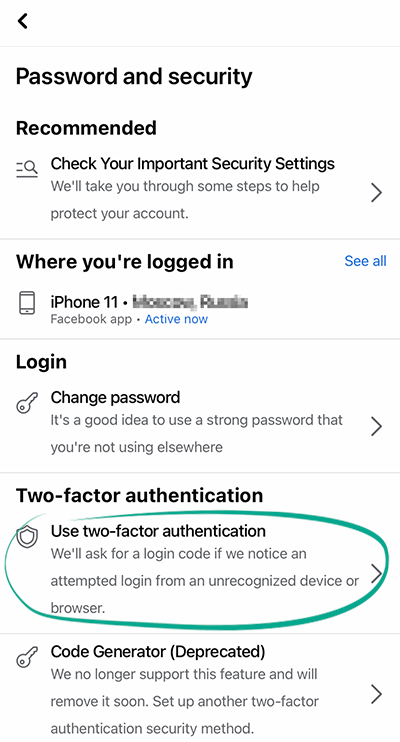This is an image of a password and security settings form on a white background with all text bolded for clarity. The form is divided into several sections, each with a bolded heading.

1. **Recommended:**
   - **Heading:** "Check your important security settings."
   - **Details:** "We'll take you through some steps to help protect your account."
   - **Visuals:** An arrow pointing towards the next section.

2. **Device Information:**
   - **Logged-in Device:** "iPhone 11 via Facebook app"
   - **Status:** "Active now"
   - **Option:** "See all" links to view other logged-in devices.

3. **Login:**
   - **Heading:** "Change Password"
   - **Details:** "It's a good idea to use a strong password that you're not using elsewhere."
   - **Visuals:** An arrow pointing towards the password change option, encircled with a thick blue pen for emphasis.

4. **Two-Factor Authentication:**
   - **Heading:** "Use Two-Factor Authentication"
   - **Details:** "We'll ask for a login code if we notice an attempted login from an unrecognized device or browser."
   - **Visuals:** An arrow guiding the user to set up two-factor authentication.

5. **Additional Security (Deprecated):**
   - **Heading:** "Code Generator (Deprecated)"
   - **Details:** "We no longer support this feature and will remove it soon. Set up another two-factor authentication security method."
   - **Key Icon:** Accompanies this section to symbolize security features.

This layout ensures users are guided through essential security settings and encouraged to enhance their account protection through strong passwords and two-factor authentication methods, highlighting deprecated features they should update.